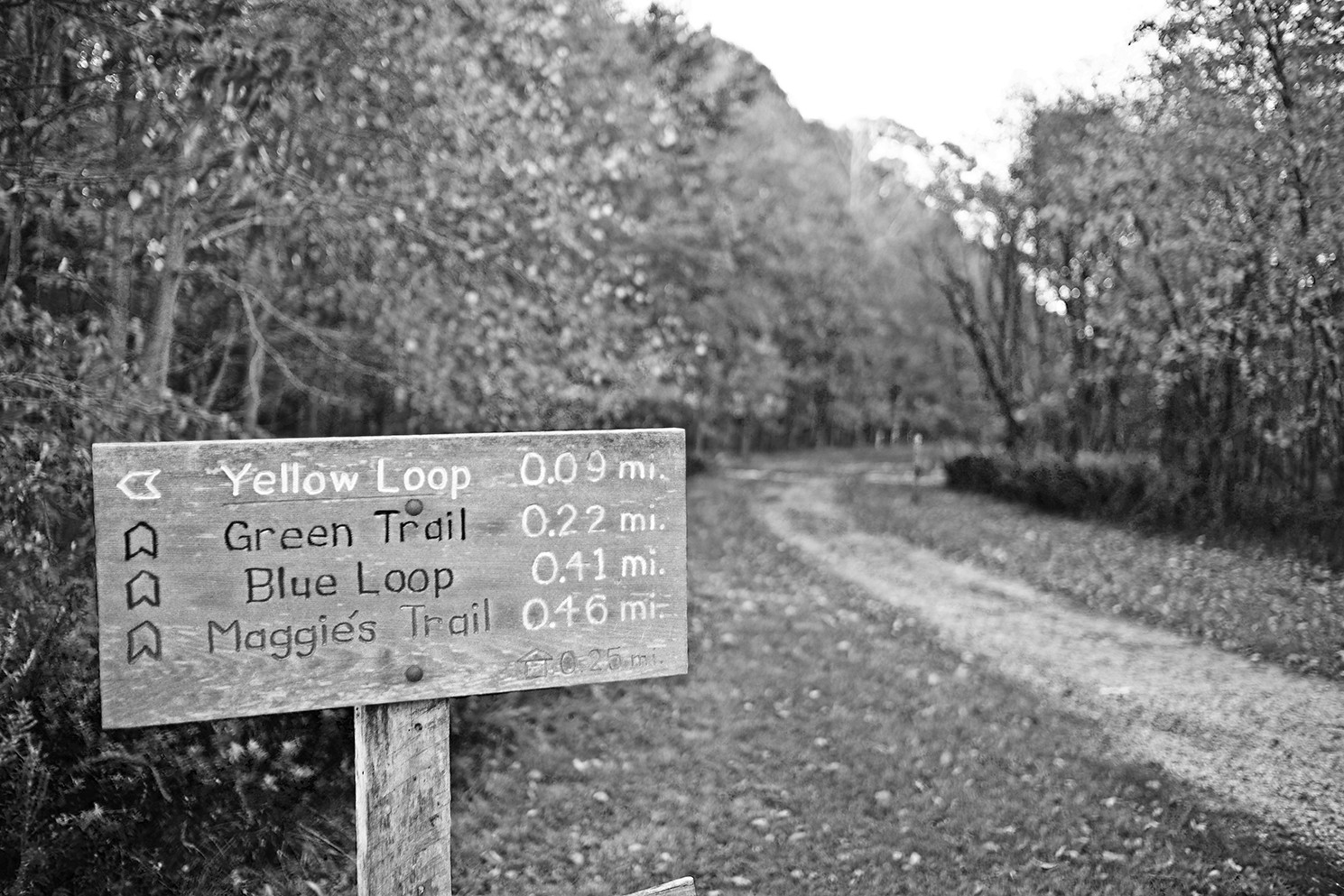The photograph is a simple yet captivating black and white image taken outdoors during the daytime, capturing a serene, horizontal rectangle scene of a nature hiking trail. The blurry background reveals a forest filled with trees, while a clearly defined, lighter path winds through the landscape, suggesting a tranquil journey through nature. Prominently placed in the left foreground is a wooden directional sign that marks various trails: the Yellow Loop, which is 0.09 miles, the Green Trail at 0.22 miles, the Blue Loop at 0.41 miles, and Maggie's Trail, the main trail at 0.46 miles. The trail, appearing wider than a typical bike path and made of even, flat gravel, seems suitable for a leisurely walk and potentially accessible for wheelchairs or walkers with canes, enhancing its inviting nature for all adventurers.